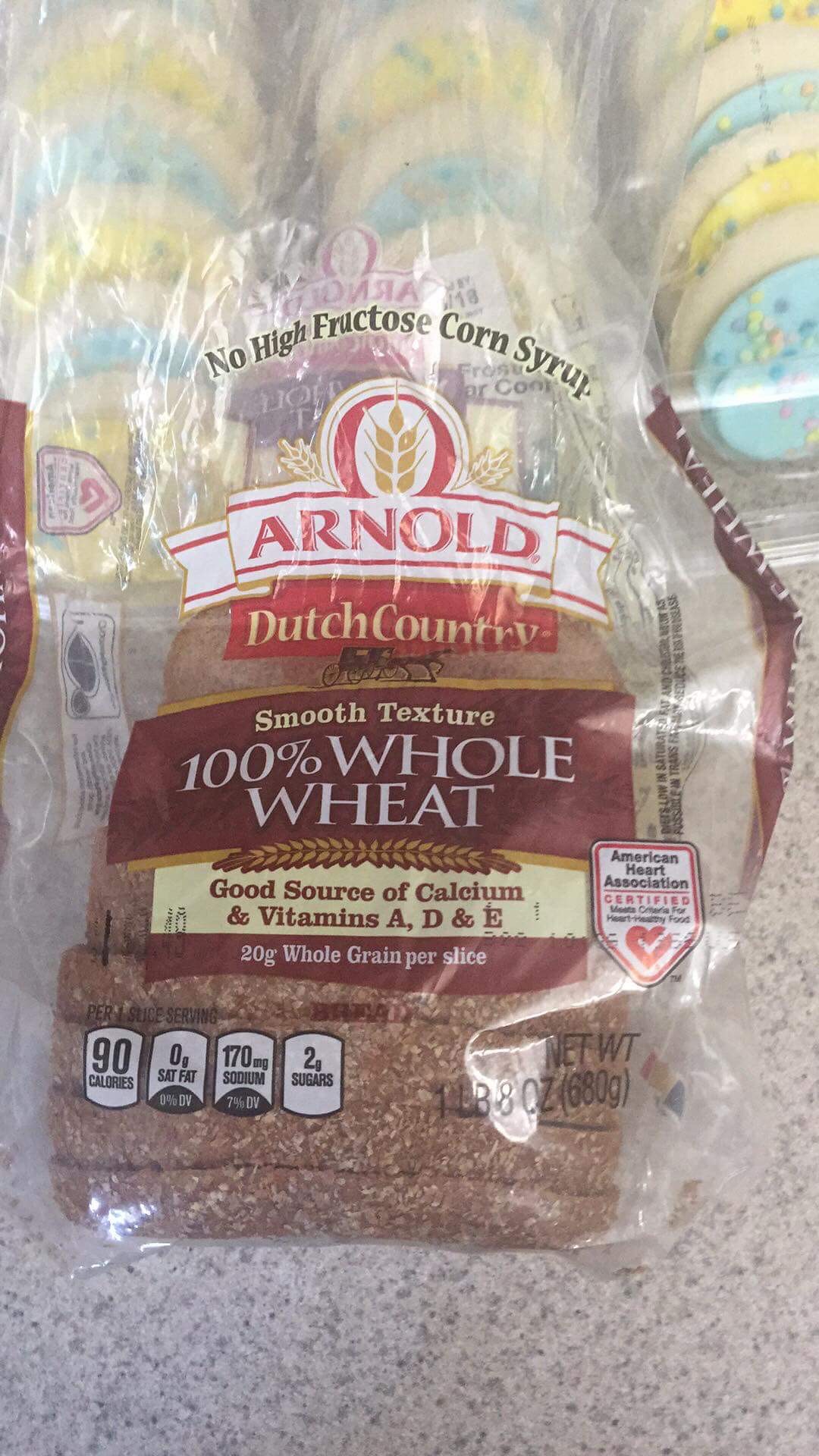The image showcases a detailed view of a marble-like surface characterized by a mix of gray, black, and white swirls, creating a visually striking backdrop. Situated at the bottom of this surface is a package of Arnold Dutch Country bread. The packaging is distinctive, with the word "Arnold" prominently displayed in red on a white banner. Below it, "Dutch Country" is written in yellow against a black background. The package also highlights several key features of the bread: 
- "Smooth Texture 100% Whole Wheat" is written in white on a brown background.
- "Good Source of Calcium and Vitamins A, D, and E" appears in brown text on a yellow background.
- "20g Whole Grains Per Slice" is indicated in white text on a brown background.
- The net weight of the bread is listed as "1 Pound 8 Ounces (680g)" in black text.

In the background, there are clear plastic containers holding an assortment of sugar cookies. Some of these cookies are adorned with blue icing and sprinkles, while others are decorated with yellow icing and sprinkles, adding a dash of color and contrast to the image.